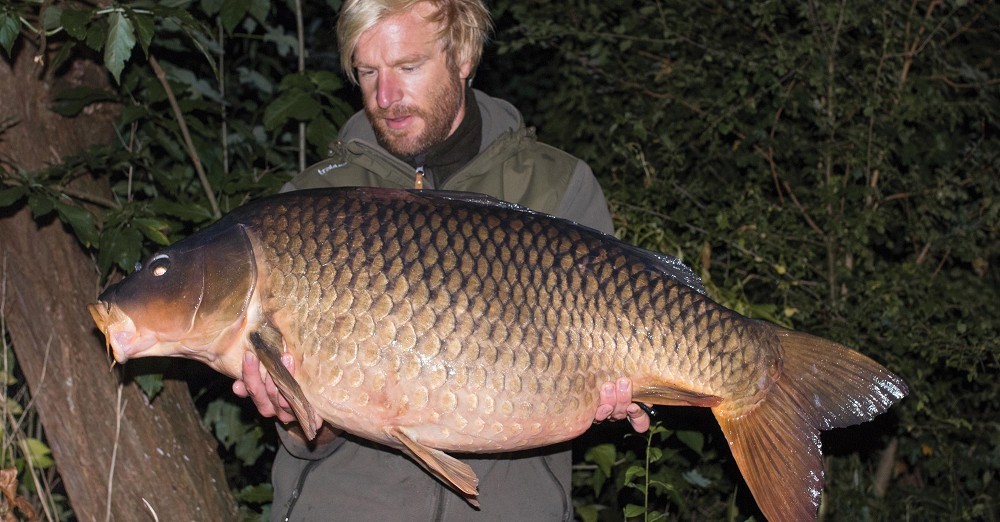A man with blonde hair, a blonde beard, and a mustache stands outdoors, clad in a gray jacket with what appears to be a black inner layer. He holds a very large fish with both hands under its belly, looking down at it in awe. The fish is predominantly muddy brown on top with intricate scale patterns featuring black lines, transitioning to a golden hue and a lighter shade on its underside. Its mouth is open, forming an O shape, and its eyes are dark. The backdrop consists of a tree trunk on the left and thin twigs with green leaves, reinforcing the natural, outdoor setting.